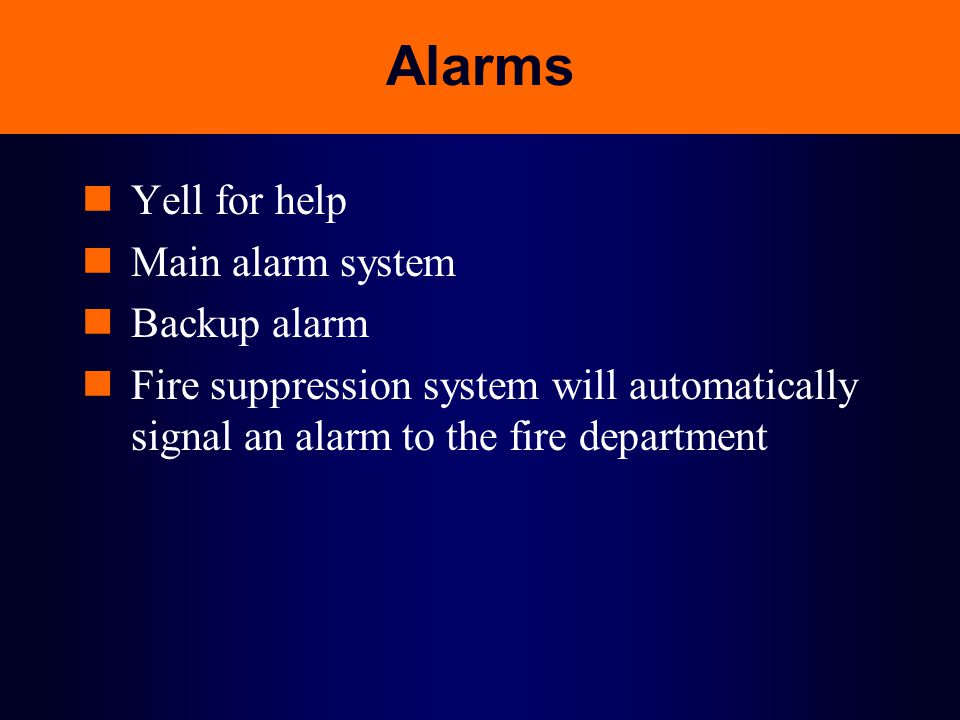The image is a poster with a header that features a vibrant orange strip at the top with the capitalized text "ALARMS" in black. The main body of the poster is a rich navy blue that darkens towards the edges, creating a gradient effect. White Times New Roman font is used for the text, which is organized into four bullet points, each marked by an orange square. The bullet points list the following instructions: "Yell for help," "Main alarm system," "Backup alarm," and "Fire suppression system will automatically signal an alarm to the fire department." The detailed layout and vivid colors suggest that this poster is likely intended as an instructional guide on how to respond in emergency situations involving alarms.